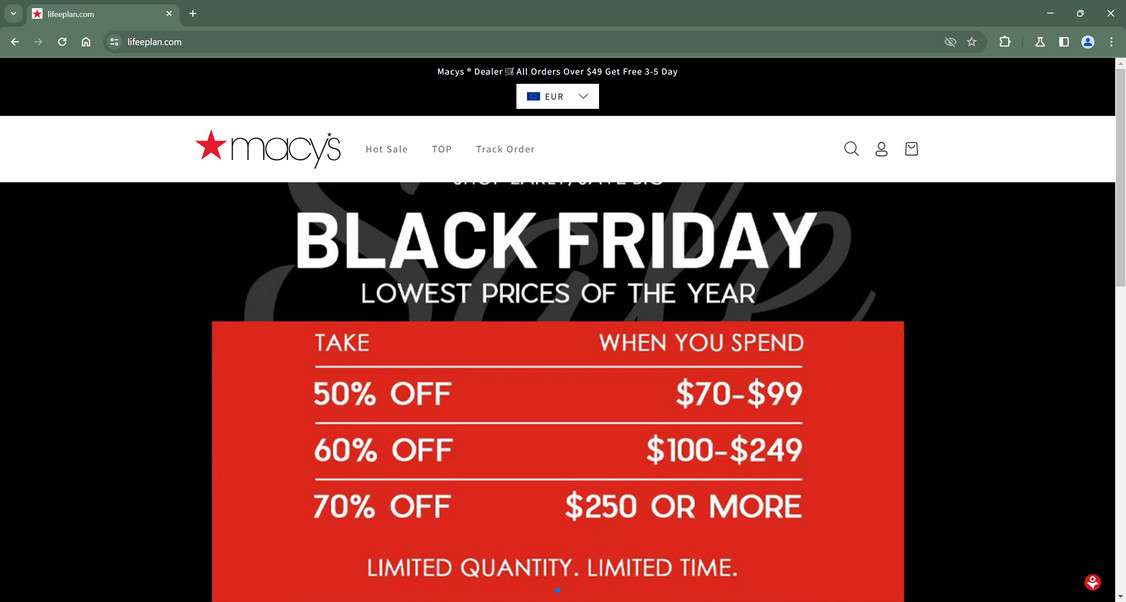This is a screenshot from a possibly misrepresented section of Macy's website taken during a Black Friday sale. The top left corner of the webpage prominently features the Macy's logo alongside its iconic red star emblem. It appears the user has navigated to this page through a site called "lifeplan.com" or "lifeeplan.com," though this intermediary step makes the layout somewhat unusual.

Directly beneath the Macy's branding, there's additional text indicating "free 3-5 day shipping on all orders over $49." A dropdown menu is available for selecting regional preferences, currently set to "Europe." The top navigation bar lists three tabs: "Hot Sale," "Top," and "Track Order."

The main content highlights Black Friday promotional deals with text proclaiming "lowest prices of the year." A sidebar on the left displays various discount tiers, detailing savings of 60%, 50%, and 70%, depending on spending thresholds ranging from $70 to $99.